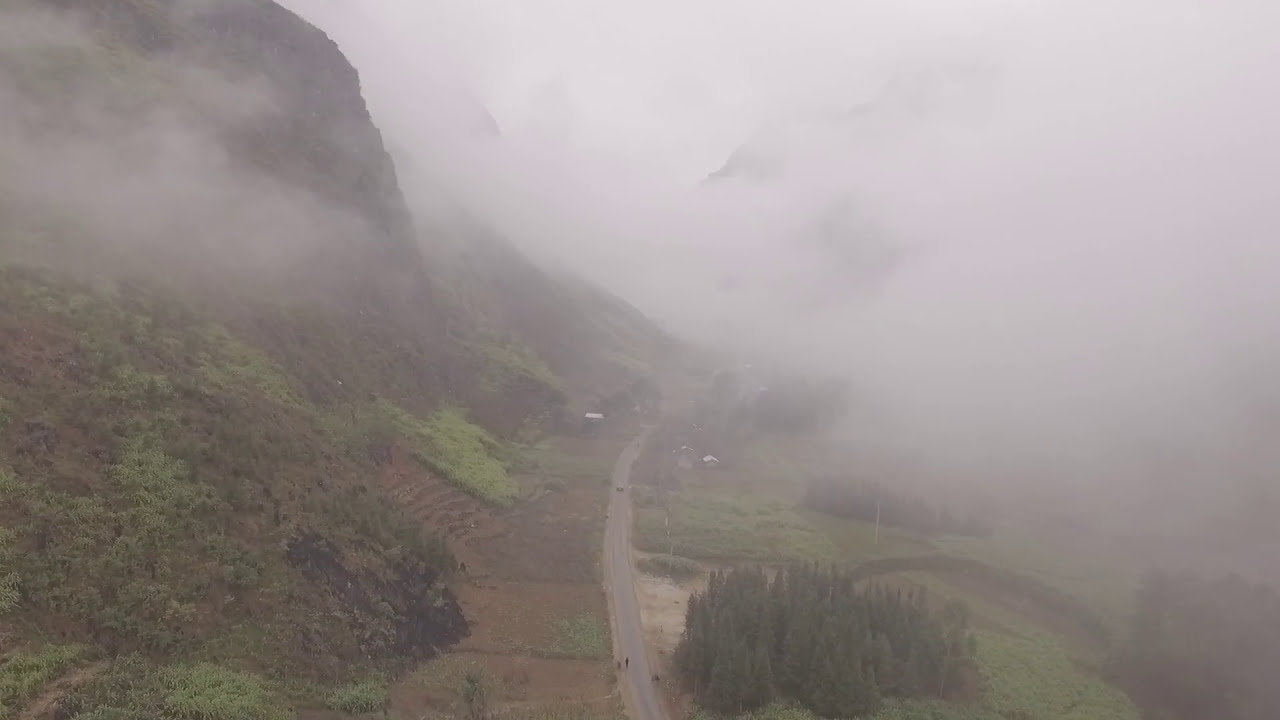This horizontally aligned rectangular image depicts an aerial view of a foggy, mountainous landscape. The upper left-hand corner features a steep, tree-covered mountainside with surrounding smaller hills. In the center right of the image, a road winds through a flattened area where some land appears prepared for cultivation. On this road, near the bottom of the picture, a car is seen driving, headed in our direction, with one or two people walking towards it. The lower right-hand side of the image is densely populated with trees. The upper right-hand corner and extending across the middle is shrouded in dense fog, rendering the sky almost invisible and blending into a blur of gray and white. Some buildings and homes are faintly visible in the background, but the pervasive fog covers much of the scene, making it difficult to see the full extent of the landscape.